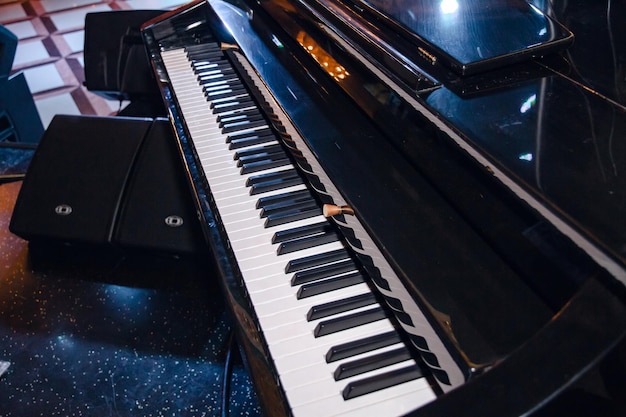The image depicts a sleek, black electronic organ situated in what appears to be a home setting. The organ features a central digital screen and a full set of white keys with black sharp keys. In front of the organ is a small, black stool. Attached to the back of the organ is a shiny, reflective screen presumably used for reading music, and appears to be computer-operated. The floor beneath the organ is tiled in black with scattered white dots, and nearby, there is a carpet adorned with geometric square patterns, adding a touch of visual interest to the room.